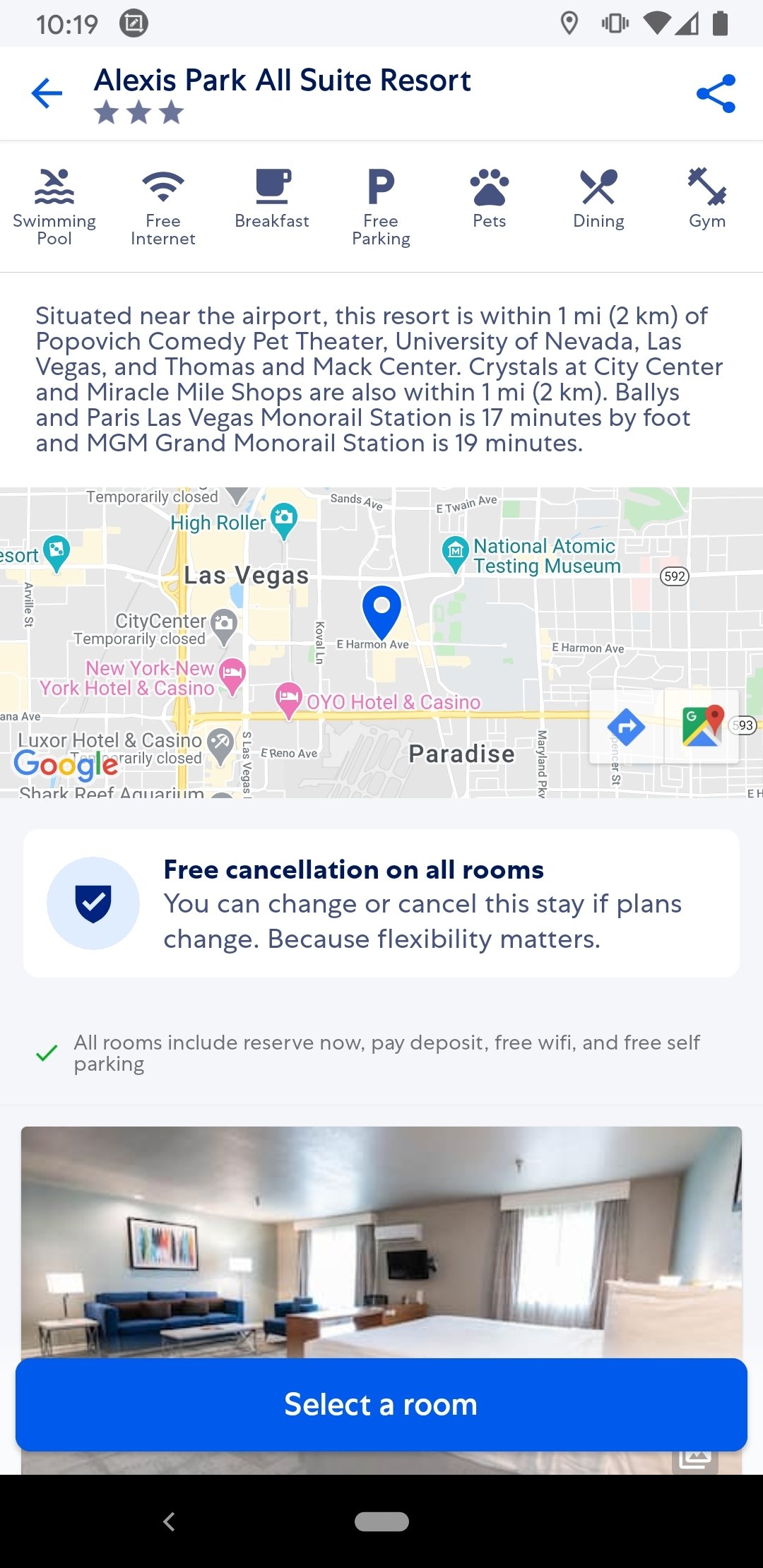Here is the cleaned-up and detailed caption for the provided image description:

---

This is a screenshot of a page displayed on a mobile phone for Alexis Park All Suite Resorts. The resort is rated three stars. Below the resort’s name, there are several icons representing the available amenities: a swimming pool, free internet and breakfast, free parking, pet-friendly accommodations, dining options, and an on-site gym. 

Beneath these icons, a description covers about six lines of text, mentioning the proximity of the hotel to the airport, emphasizing its convenient location. The resort is situated in the Las Vegas area, specifically in South Las Vegas near Paradise. A map is displayed below the description, highlighting the resort's location with a blue location bubble.

Following the map, a white banner indicates that all rooms come with free cancellation, marked by a check. Accompanying details specify that all rooms offer "reserve now, pay deposit" options, free WiFi, and free self-parking, each feature confirmed with a green check.

The last section shows an image of a hotel room, featuring a couch against the back wall, two large windows with a mounted TV in between, a small wooden desk, a coffee table, a lamp, two beds, and an end table. Above the image, there is a blue "Select a Room" button. At the bottom of the screen is a black header with a left-pointing arrow.

---